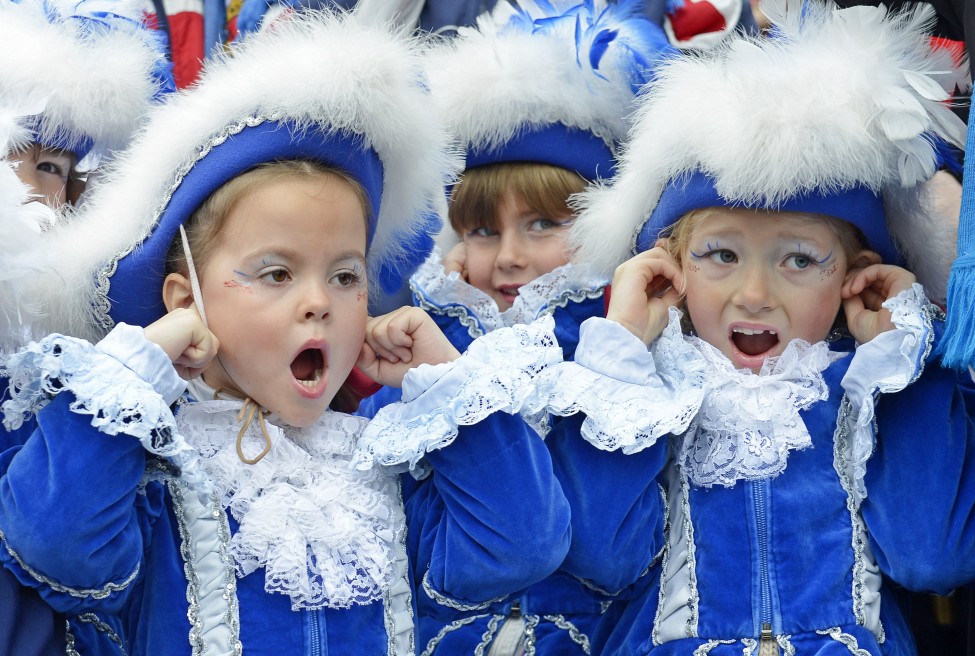In this detailed photograph, four little girls, approximately five years old, are dressed in elaborate blue and white uniforms reminiscent of 1700s attire, possibly indicating their participation in a cultural festival. The girls wear long-sleeved blue shirts adorned with white fringes at the neck and wrists and feature two white strips down the front. They all sport matching blue hats topped with white feathers. The girls are visibly reacting to a loud noise, as each one has her fingers in her ears and their mouths open, seemingly yelling or expressing discomfort. The girl in the center has blonde hair and appears particularly noticeable for her open mouth and direct reaction to the sound. To her right stands another girl with light brown bangs who is similarly dressed and looking toward the camera. A fourth girl is partially obscured in the background, contributing to the sense of a larger crowd. The image captures their expressions vividly, with hints of light face paint around their eyes, adding to their festive appearance. The scene suggests a noisy outdoor setting, with the children distracted by something off-frame.